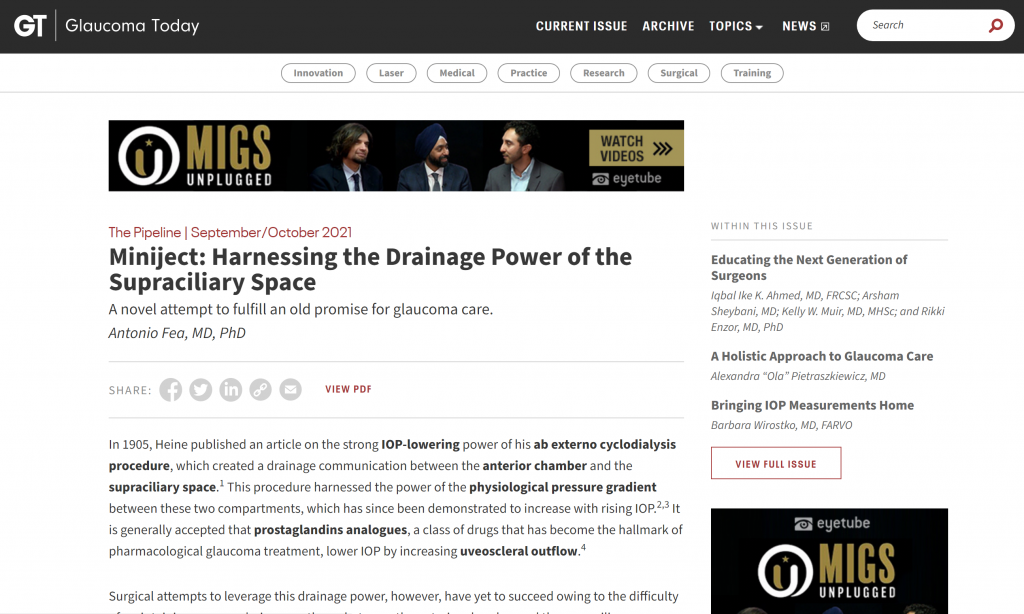Screenshot of the "Glaucoma Today" Website

At the top of the website is a sleek black banner. In the top-left corner, "GT" is prominently displayed in large white letters adjacent to a vertical white line. The words "Glaucoma Today" are written in smaller white letters immediately to the right of this line. Further along the right side of the banner, you find navigation options labeled "Current Issue," "Archive," "Topics," and "News," all in white letters, followed by a search bar at the far right.

Directly below the black banner are oval-shaped menu buttons against a white background. These buttons, outlined in gray with gray text, list categories such as "Innovation," "Laser," "Medical," "Practice," "Research," "Surgical," and "Training."

The main section of the webpage showcases a large advertisement banner at the top, titled "MIGS Unplugged," featuring a photograph of three men. The ad encourages viewers to "Watch Videos on iTube." Beneath the ad, the current issue information is presented in red text, highlighting "The Pipeline, September/October 2021." Directly below this is the article headline, "Miniject: Harnessing the Drainage Power of the Suprachoroidal Space," followed by author information, sharing options, and a link to view the PDF version of the article.